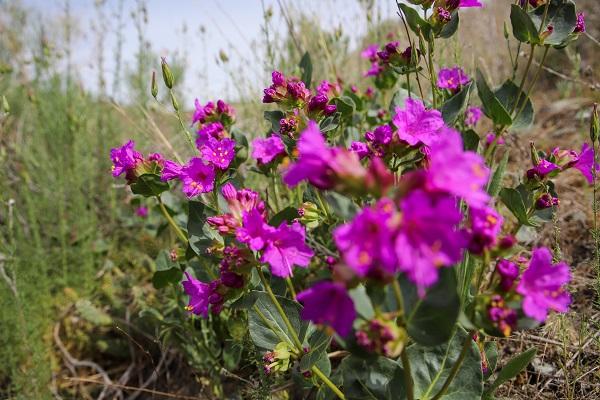This professional close-up shot captures a vibrant field of small purple flowers, possibly violets, in full bloom. The scene is bathed in sunlight under a bright blue sky, emphasizing the natural beauty of the wild landscape. Tall, lush green grass surrounds the flowers, interspersed with sticks, brush, and some weeds, highlighting the untamed nature of the setting. Some flowers are prominently featured in the foreground, although slightly out of focus, drawing attention to the mid-range bloom that is sharply in view. The petals of the flowers reveal delicate yellow seeds within, adding a touch of intricate detail. The background, filled with more greenery, blends into the sky, creating a serene and expansive horizon. The overall image showcases a thriving, uncut meadow teeming with life and color.